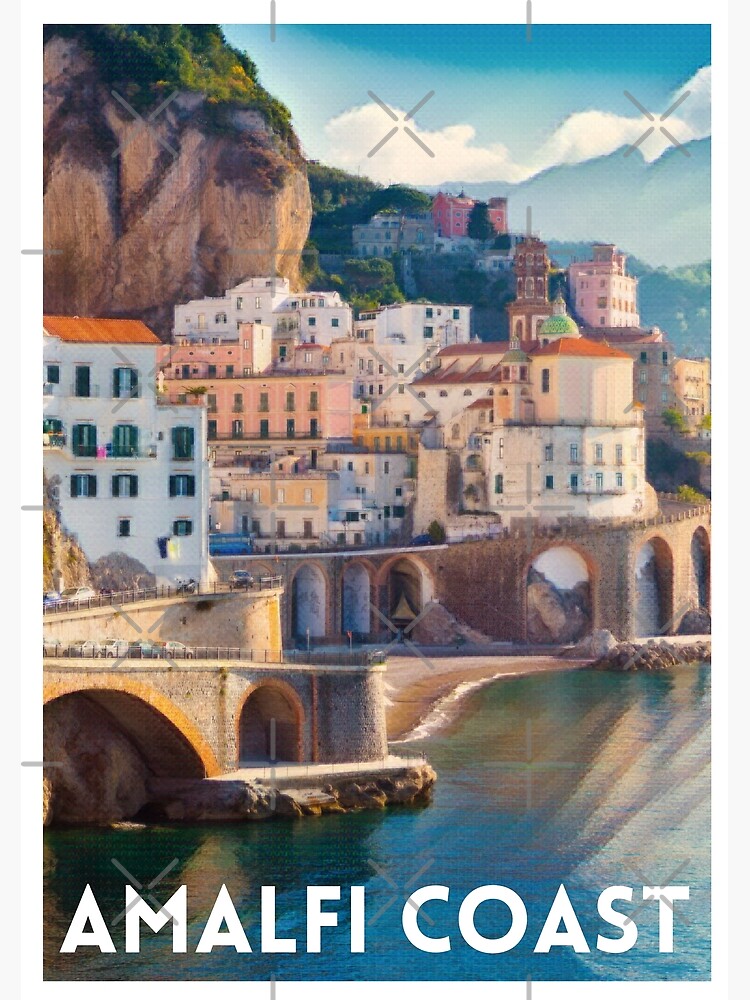This poster, titled "Amalfi Coast" in large white letters at the bottom, features a vividly painted scene reminiscent of an Italian coastal village. At the top of the image, a blue sky with white clouds stretches over a rustic village set against majestic green-topped mountains. The village itself cascades down to the waterfront, where a small beach meets the ocean. Multicolored buildings in shades of white, pink, peach, and brown are interspersed with vehicles parked along a stone wall that borders the town. These buildings include arched doorways and windows, some appearing to be built into the mountainside, enhancing the old-world charm of the scene. The left-hand side of the image reveals a tunnel with a yellow opening, adding an element of intrigue. Overall, the entire scene exudes a picturesque and idyllic coastal ambiance, beautifully capturing the essence of the Amalfi Coast.